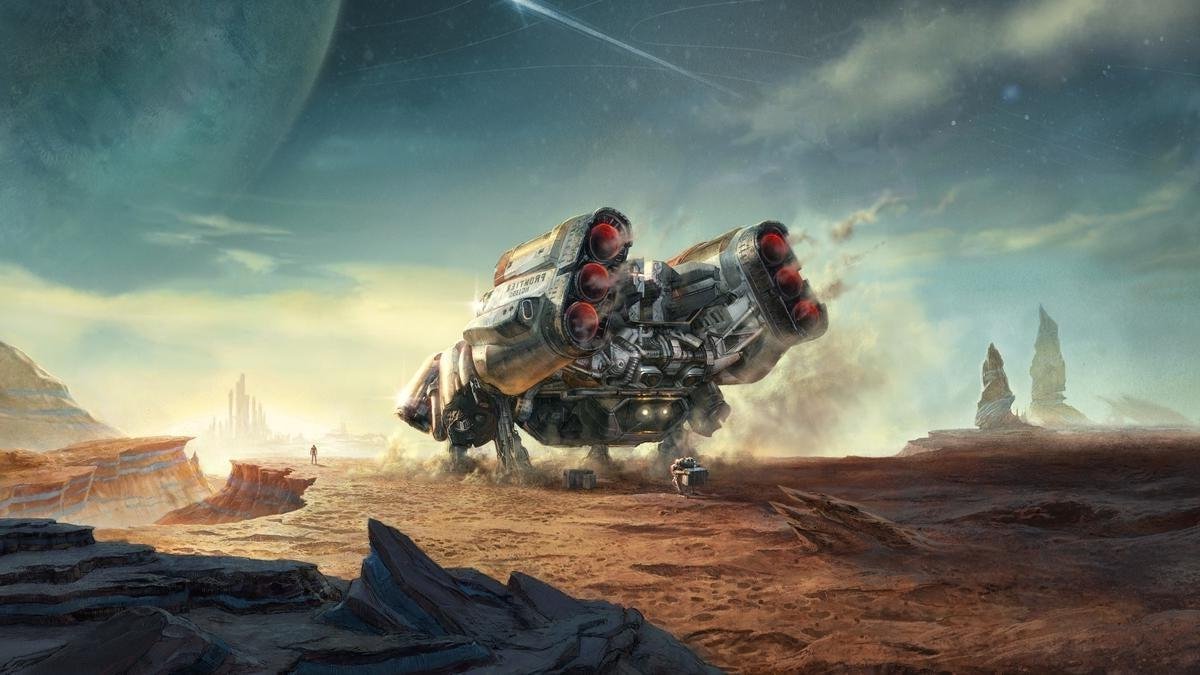A stunning, futuristic landscape illustration captures a dramatic scene of a robotic, crab-shaped spaceship landing on a rocky, alien terrain. The mechanical spacecraft, with its elliptical dark metal body resembling a saucer, stands poised on four segmented legs, each ending with wide claws featuring three torpedo-like rockets emitting orange flames and smoke. Dust rises around its footing, creating the impression of a recent touchdown. The landscape is dominated by sharp, pointed rock formations and a sheer cliff to the left, where a lone figure stands near the edge, perhaps observing the scene or contemplating the distant, glowing cityscape with its unique, tall structures. Above, a vast golden moon hangs in a blue, partly clouded sky, casting a warm light over the entire area. The city, bathed in golden sunlight, glimmers on the cusp of the horizon, adding an element of advanced civilization to the otherwise rugged and wild terrain. The illustration, rendered in vibrant colors, seamlessly blends elements of fantasy and science fiction, evoking a sense of exploration and the unknown.